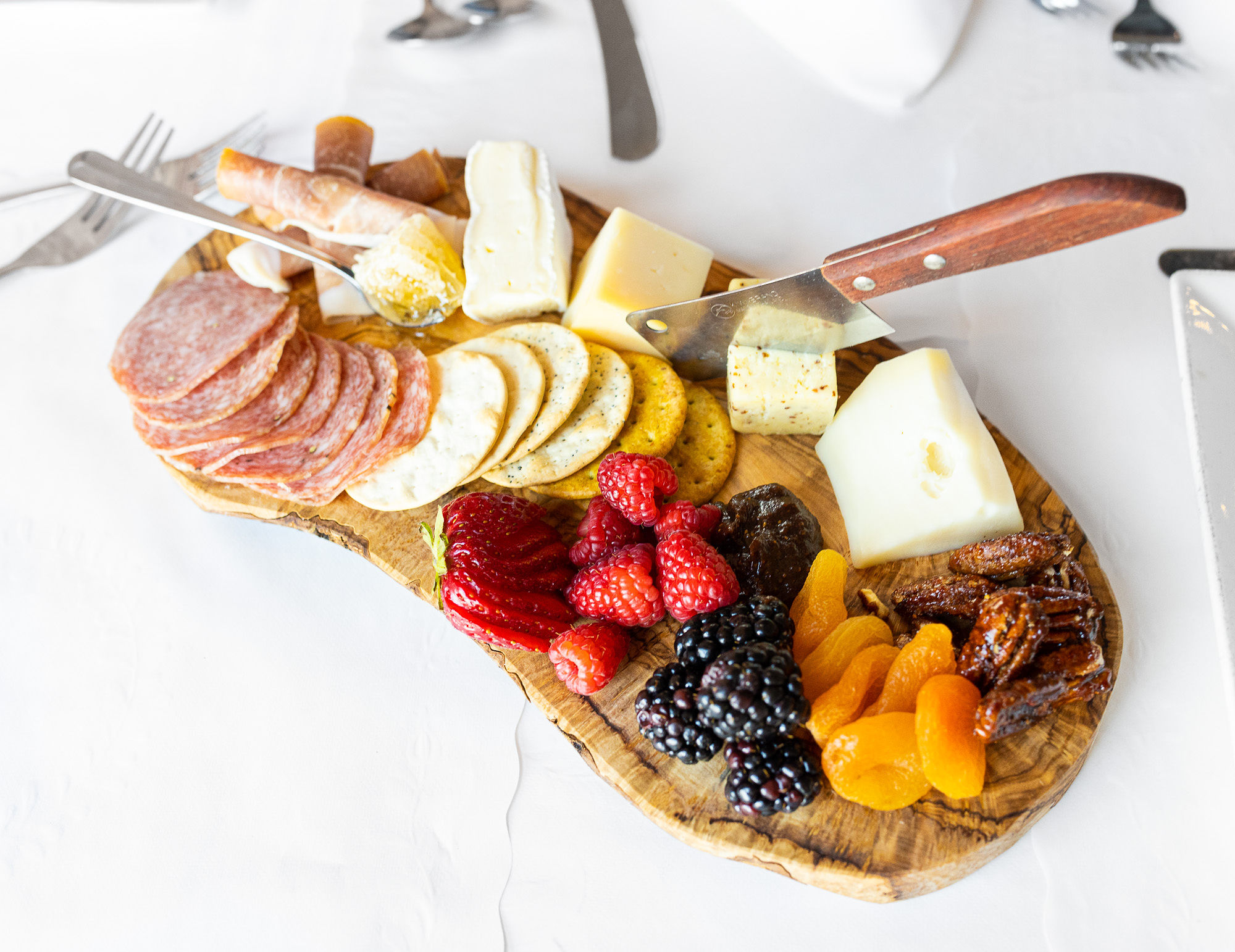This image features a tantalizing charcuterie spread artfully arranged on an organically shaped wooden chopping board. The board showcases a variety of delightful food items, including sliced salami and another type of ham, an assortment of crackers, a sliced strawberry, six raspberries, four blackberries, five dried apricots, a small handful of walnuts, and a prune. A selection of cheeses—ranging from soft to hard varieties—adds to the rich variety of the spread. Accompanying the food are a small cheese knife and a serving spoon, ready for use. The scene is set on a white table, which has scattered cutlery such as forks and spoons in the background, along with a square white plate situated at the edge. The arrangement is modern and clean, looking exceptionally appetizing and colorful, making it perfect for one or two people to share. The overhead perspective highlights this refined and elegant presentation, inviting anyone to indulge in its carefully curated selection.